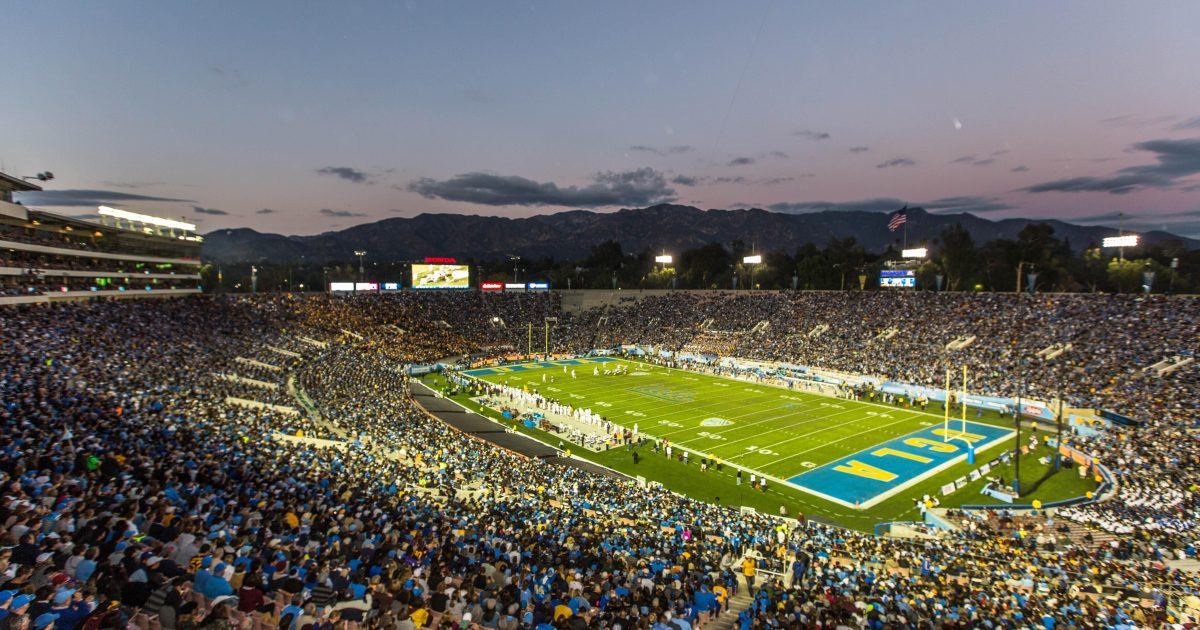This night-time photograph captures the vibrant atmosphere of a football game at a stadium filled with thousands of spectators. The field, prominently displaying "UCLA" in yellow and blue in both end zones, is in the lower right part of the image, accented by bright stadium lights that illuminate the scene. The bowl-shaped stadium is teeming with a sea of blue and gold-clad fans, matching the team's colors on the field. Beyond the crowd, various screens and advertisements light up the outskirts of the stadium, including a noticeable bright billboard on the left side. Behind these, a field house building is visible. The sky, painted in shades of blue and light purple, forms a picturesque backdrop with silhouetted mountains and scattered clouds. An American flag can be seen on the right side, further enhancing the patriotic spirit of the event.